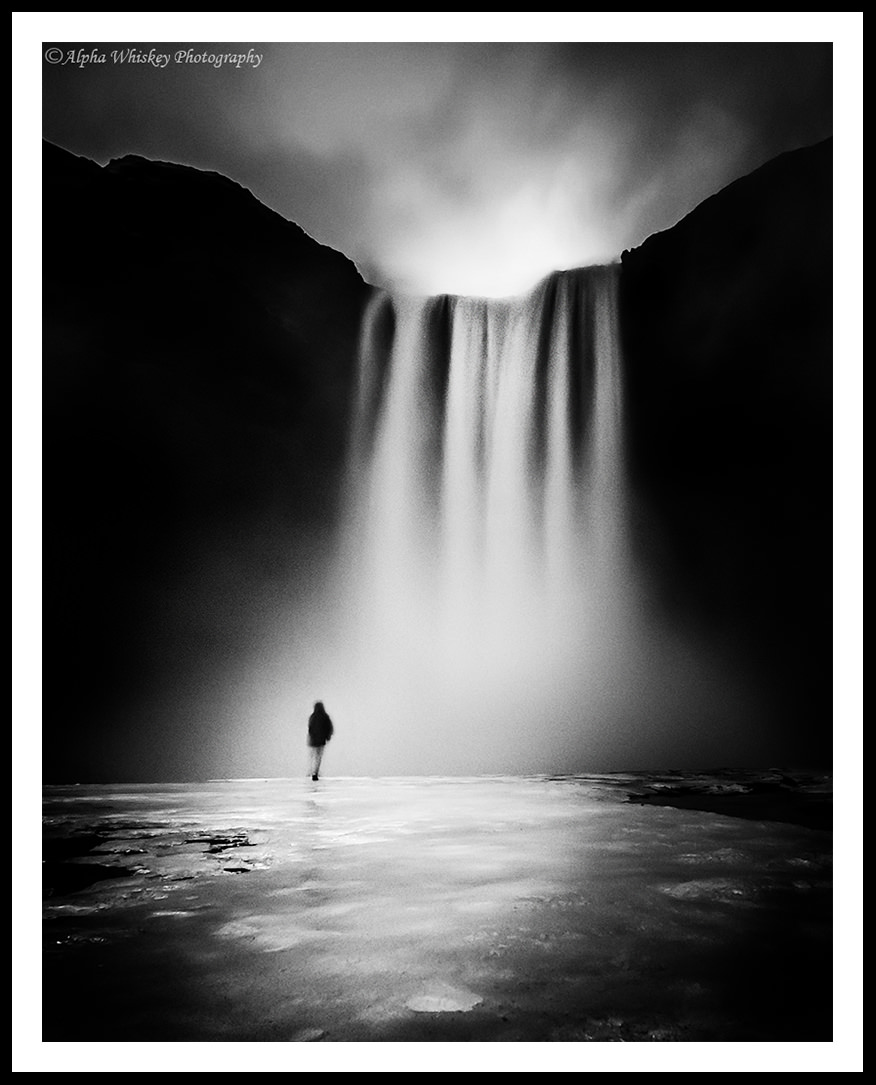The photograph is a vertically aligned, black and white image, elegantly framed with a thin black outer border and a thicker white inner matte. In the upper left-hand corner, there's a copyright symbol marked "Alpha Whiskey Photography." The photograph features a large, striking waterfall that descends from a silhouetted cliff, which dips slightly in the middle where the waterfall cascades. The sky above the cliff is a blend of gray and white, imparting a cloudy, smoky appearance.

In the foreground, at the bottom of the image, a person stands on smooth, wet land, facing the majestic waterfall. The individual, donning a dark jacket and light-colored pants, appears small in comparison to the grand scale of the waterfall, emphasizing its impressive height, estimated to be around 50 feet. The water appears as vertical streaks of light gray and white, creating a misty, ethereal effect as it plunges down. The ground around the figure mirrors the same grayscale tones, with darker areas in the lower corners of the image. The composition captures a sense of solitude and awe-inspiring natural beauty.